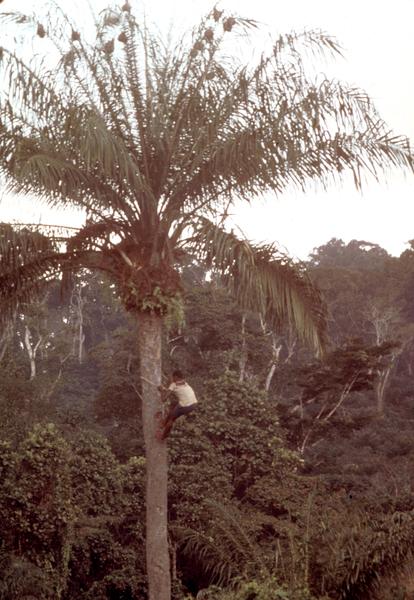The image depicts a faded, vintage outdoor scene set during the daytime, characterized by a clear white sky. At its center stands a towering palm tree, distinctly taller than other various-sized trees surrounding it in a jungle or rainforest-like setting. This central palm tree, which appears to have minimal leaves and a section where a branch has been neatly cut off, has a long, slender trunk. Climbing this tall tree is a man using a rope for support. He is dressed in a white t-shirt and black pants, and he appears to be barefoot. The man seems intent on reaching the top, possibly in search of coconuts. The overall color palette of the image is muted, emphasizing the aged and remote atmosphere.